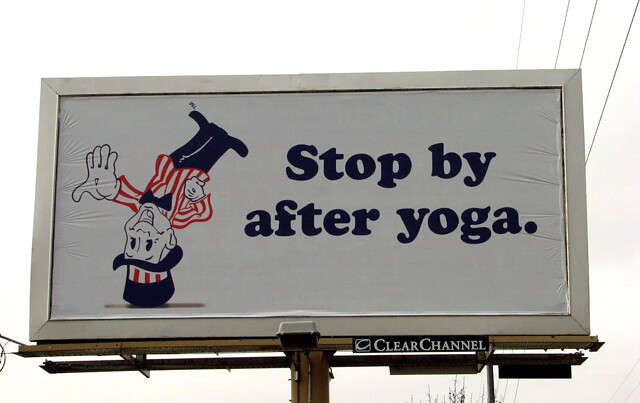The image showcases a detailed billboard standing on a brown steel pole platform, equipped with a black and white light spotlight at the base. The billboard itself has a white background and a white frame. Dominating the scene is a simplistic cartoon figure, reminiscent of Uncle Sam or a big top announcer from the 1920s or 1930s, dressed in a vintage outfit. He wears a top hat adorned with red and white stripes, a shirt with red stripes, black pants or boots, and a red and white bow tie. The figure is depicted upside down with one hand on his hip and the other stretched out towards the viewer, his palm facing outward and fingers pointing downwards, all while smiling. To the right of the caricature, bold text reads "Stop by after yoga." At the bottom of the billboard is the Clear Channel logo, indicating the owner of the billboard.